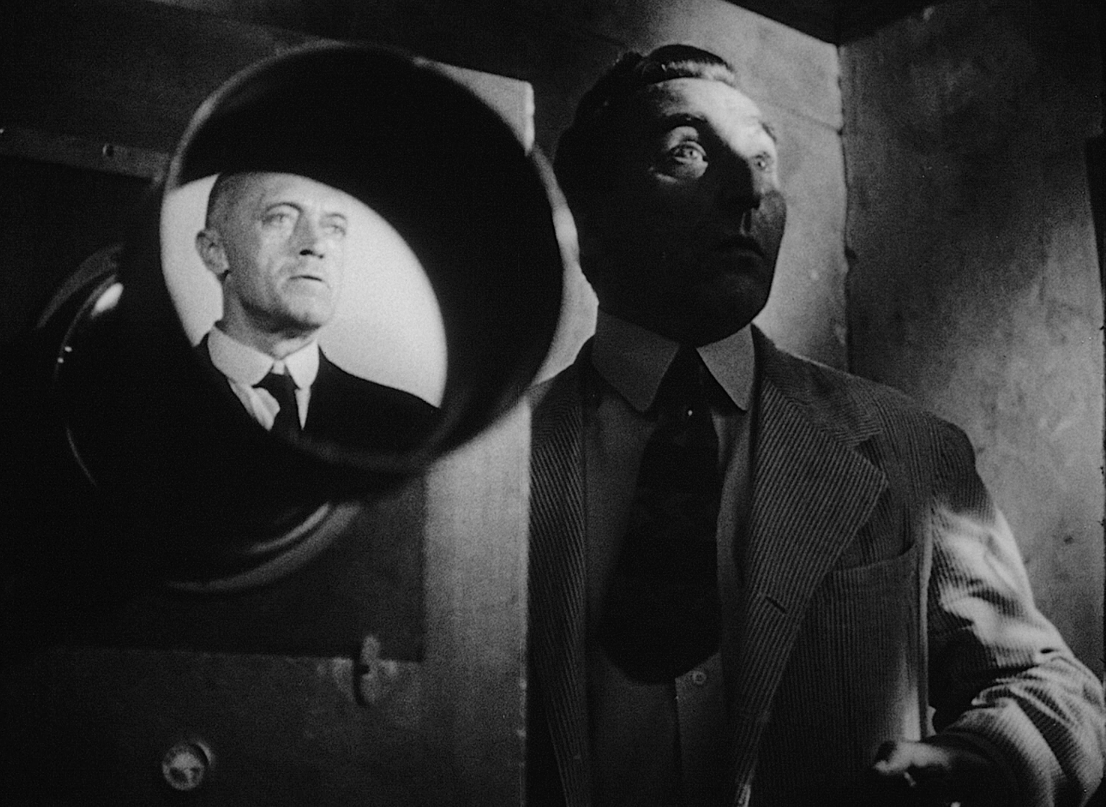This black-and-white photograph captures a tense moment from the 1946 film "The Stranger." Set in a dimly lit, dungeon-like room with rough rock walls, the grainy image exudes an aura of suspense and foreboding. Centered in the frame is a Caucasian man with his hair slicked back, dressed in a pinstripe suit, tie, and a white collared shirt. His eyes are wide open, staring ahead with a mixture of shock and surprise. 

To his right, and our left, stands an enigmatic machine that resembles a projector. Intriguingly, within the lens of this projector, the face of an older man is visible. This man, similarly dressed in a white shirt, tie, and dark blazer, appears almost ghostly, adding to the enigmatic and chilling atmosphere of the scene. The film's vintage angle and the compelling expressions captured make this a particularly striking and memorable image from classic cinema.